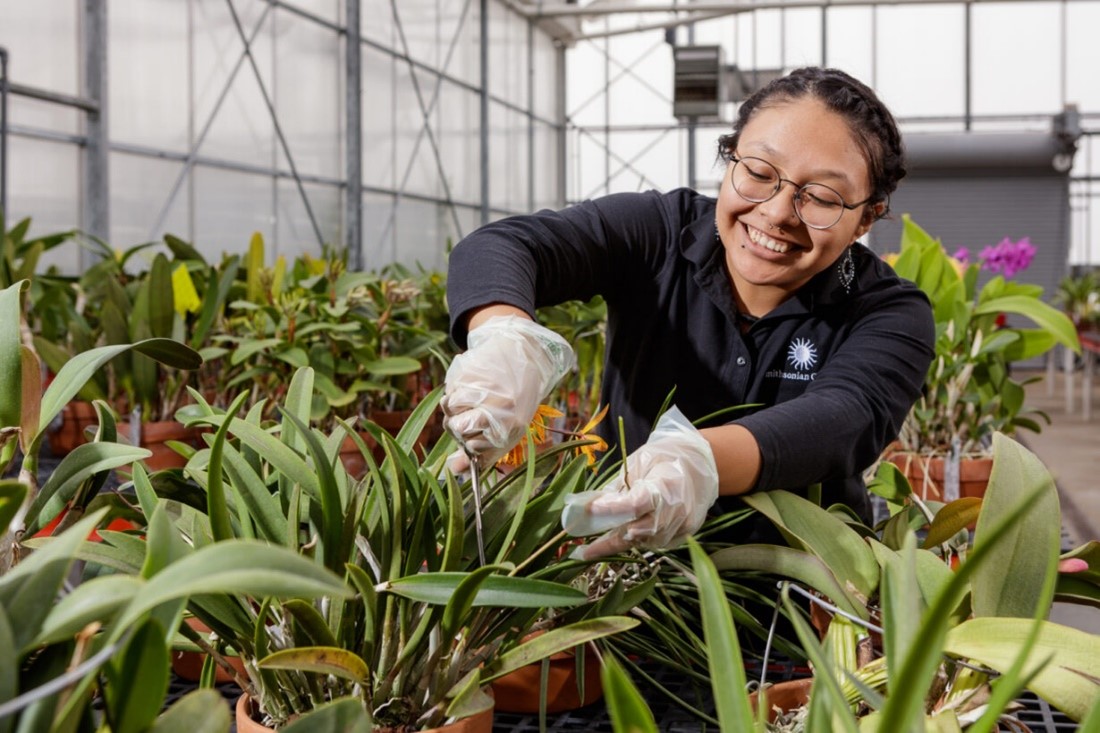The photograph captures a smiling young woman with slightly tan skin, wearing wireframed glasses and brunette hair pulled back. She is dressed in a navy button-up shirt adorned with a light blue sun emblem and some partially obscured text, possibly reading "Smithsonian Collegiate." She has on clear plastic gloves and is engaged in trimming plants with a metal tool, bending over pots of lush greenery. Surrounding her are windows of a spacious, multi-story greenhouse, diffusing natural light throughout the scene. Behind her, there are vibrant floral accents, including purple-pink flowers near her right shoulder and an orange-yellow bloom near her hands. The scene is filled with green foliage and long, frondy leaves, creating a serene and industrious gardening atmosphere.